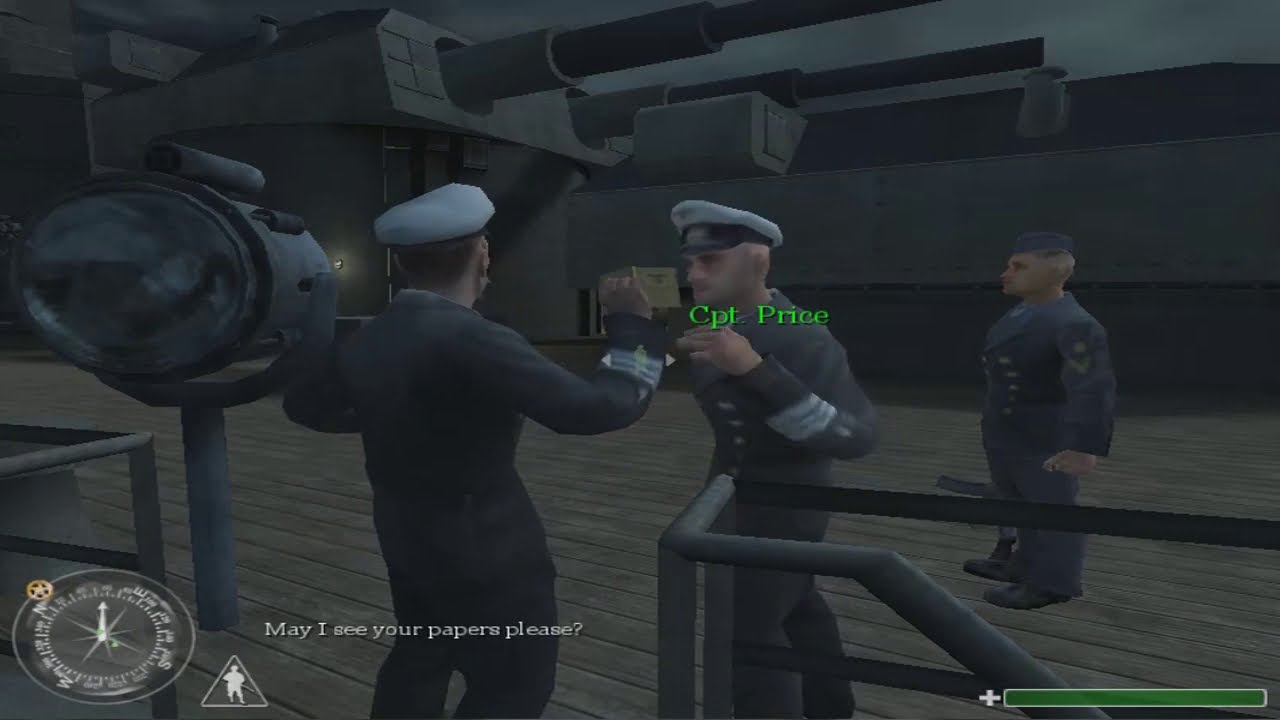This is a detailed screenshot from a video game showcasing three sailors on the deck of a Navy battleship. The ship, with its large, imposing gun turrets positioned at the top center of the image, seems prepared for battle. The deck beneath the sailors is made of wooden planks, displaying the worn look of a seasoned vessel. The overall ambiance is dark and dreary, casting a somber tone over the scene.

In the middle of the deck stands a man in a gray suit and captain’s cap, identified by the green text above him as "Captain Price." To his left are two sailors in white caps likely indicative of their higher rank, appearing to be on the verge of an altercation. The text "May I see your papers please" is displayed at the bottom of the screen, suggesting an interaction or command.

Farther to the right, a lower-ranking officer in blue stands at attention, also facing left, contributing to the apparent tension among the men.

On the left side of the image, a large spotlight or magnifier is visible, adding to the ship’s equipment arsenal. A sturdy metal railing surrounds the deck, enhancing the realism of the battleship's structure. The utility of the ship is further signified by the navigational compass at the bottom left corner of the screen and a green health bar gauge at the bottom right. This meticulously crafted scene effectively immerses the viewer in its wartime setting.